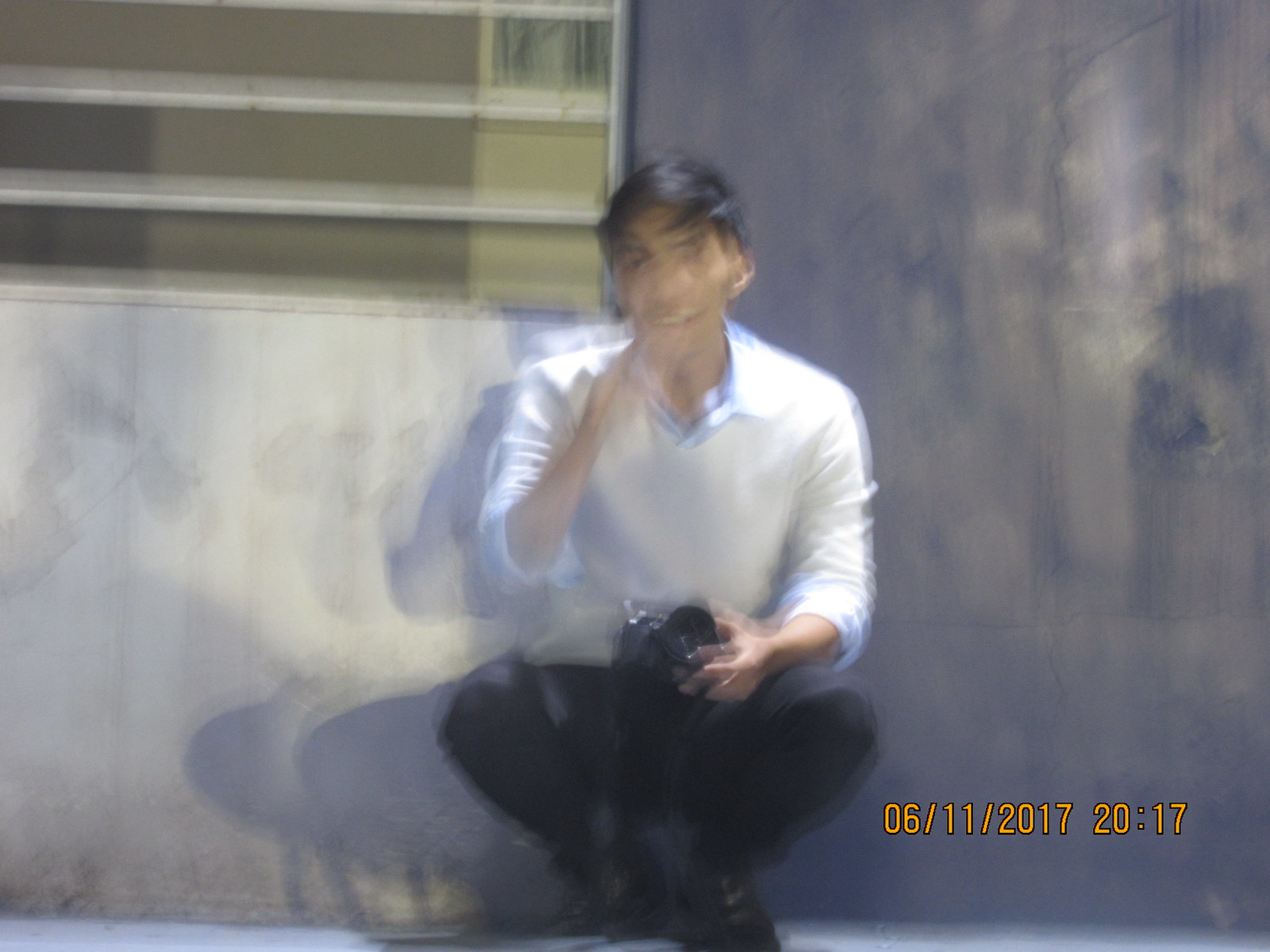This is a blurred photograph of a man with black hair, dressed in a white dress shirt unbuttoned at the collar, black slacks, and black shoes. He is squatting down, bending his knees and looking straight into the camera, while holding a black camera in his left hand. His right hand is lifted towards his mouth, suggesting he might be taking a smoke break. The background consists of a concrete wall with a small portion of a window with white horizontal lines, and a shadow cast by the man. There is a timestamp in the bottom right corner in orange text, which reads 06-11-2017 20:17, indicating the photo was taken on June 11, 2017, at 8:17 PM.